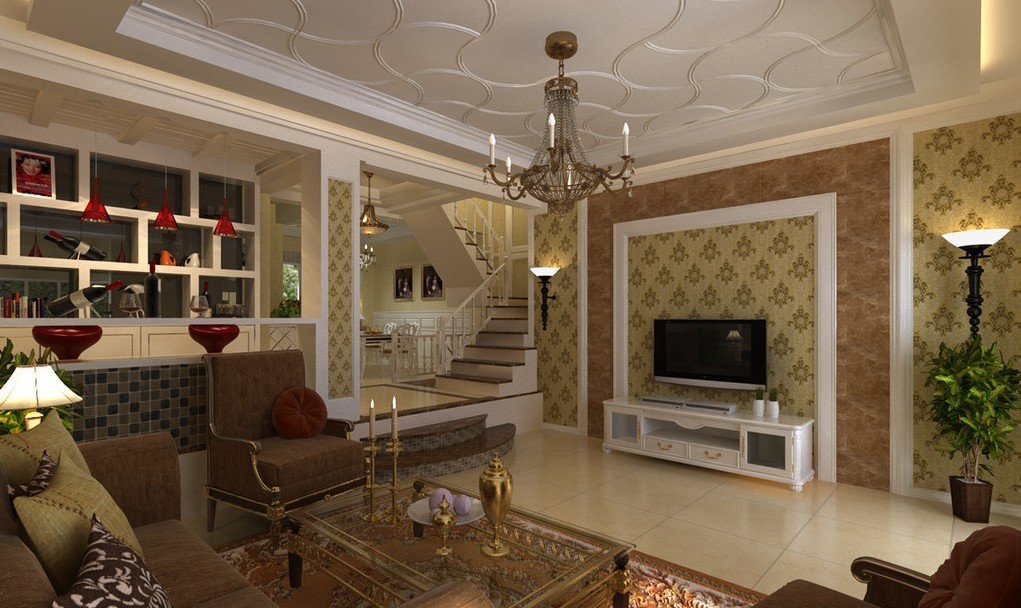The photograph depicts a spacious, elegant living room characterized by a blend of modern and classic decor. Central to the room is a large TV mounted above a long, white rectangular table with drawers, accented by gold trim. The TV and table are set against a backdrop of brownish-tan wallpaper segmented into different sections. 

On the white ceramic floor, there is a prominent oriental carpet situated in the foreground. To the left, a cozy arrangement of seating includes a brown sofa and an armchair, both with gold highlights, accompanied by another armchair in the lower right-hand side. These are positioned around a central coffee table adorned with gold candelabras, vases, and candles. 

A chandelier with intricate detailing hangs from the decorated white ceiling, providing a touch of grandeur, while additional wall lamps contribute to the ambient lighting. 

In the background, toward the left, white shelving units display wine bottles and photographs, enhanced by red barstools nearby. The room extends further with a visible stairway centrally located, leading to other parts of the house. White moldings along the walls and ceiling tops frame the entire scene, adding to the room’s sophisticated charm.